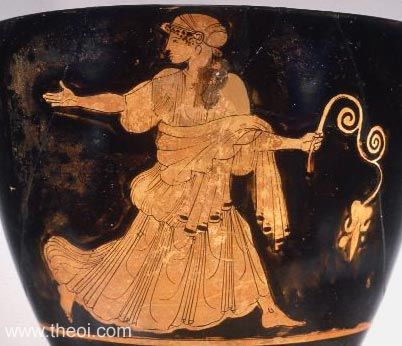This image depicts an ancient, decorative pottery piece, likely a cup or vase, showcasing a dark, distressed brown surface with a single gold ring around its base. The pottery is adorned with an intricate gold depiction of a figure dressed in elaborately etched robes. The figure, tan in color, is captured in a dynamic pose, walking barefoot and making a dramatic turn to look behind them, with their head turned to an exaggerated degree. One hand, extended forward, holds a long, coiled wand, possibly a flowering plant, with the lower portion of the plant hanging down and faintly resembling an owl. The figure wears a scarf draped over their shoulders and part of their waist. The image contains a reference to a website, www.theoi.com, at the bottom, suggesting where the pottery can be found or researched further.